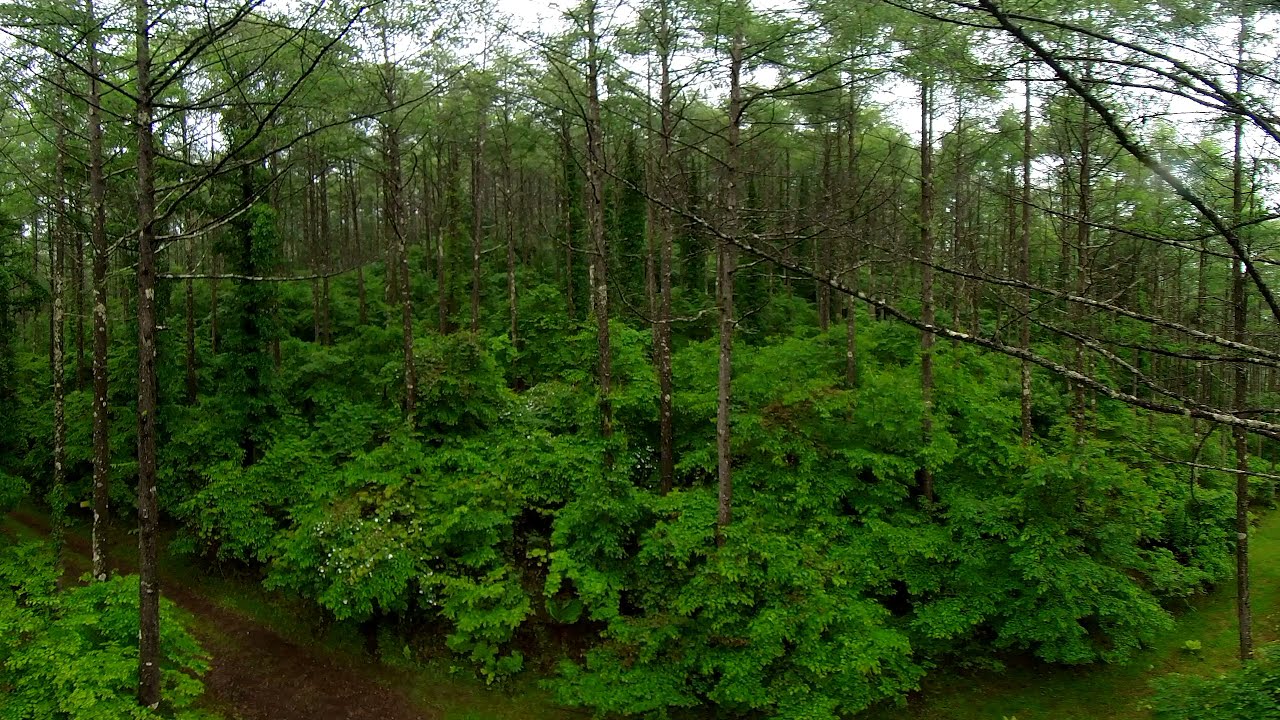This image captures an outdoor, mid-range view of a vibrant forested area. The lower half of the photograph is dominated by verdant, lush greenery, including bushes and ferns with neon green leaves that seem almost unnaturally bright, suggestive of photo manipulation. These smaller plants are interspersed with a layer of shorter trees that appear to overrun the forest floor with their abundant, vibrant leaves. The upper portion of the image is characterized by taller trees with thin, branch-like trunks that support sparse, leafless treetops, some of which appear diseased with white spots. Amidst this vibrant green foliage, a brown dirt pathway meanders through the forest, located towards the left side of the image. Blue sky, streaked with partial clouds, peeks through the uppermost fifth of the photograph, providing a backdrop to the dense greenery below.